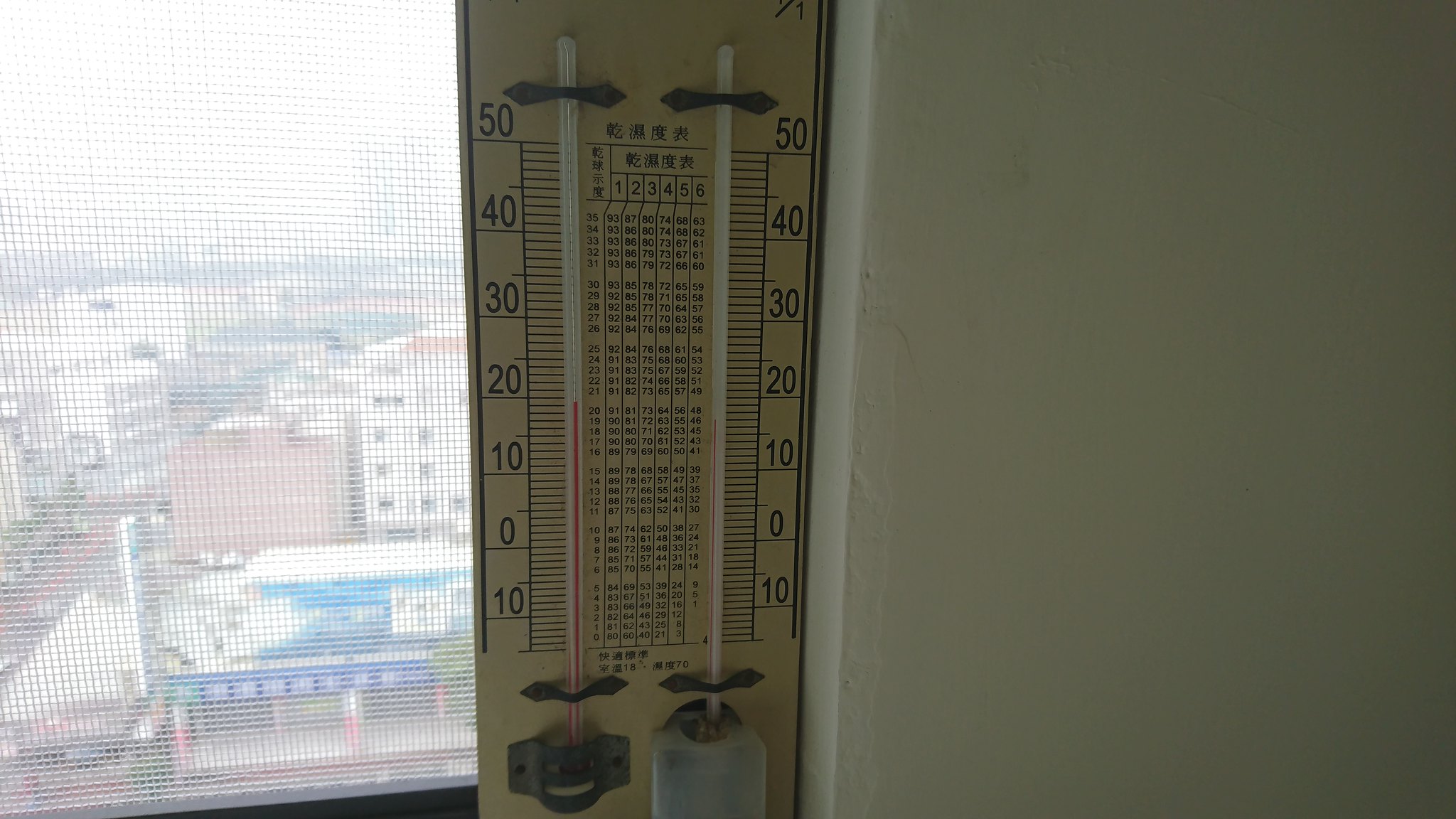The image features a thermometer positioned inside a high-rise apartment, overlooking a cityscape. The thermometer itself is brown, with markings in what appears to be Asian script, suggesting it may have been manufactured or used in an Asian context. The thermometer has dual mercury tubes, one in a dark red and the other in a lighter red hue, with identical numerical readings on both sides.

The background visible through the window adds context to the setting. The window’s screen slightly distorts the view but does not obscure the visibility of surrounding buildings and street activities. Below, one can see rooftops of adjacent buildings, indicating a multi-story urban environment. Prominent in the view is a turquoise-colored warehouse and what seems to be a train station across the street, identifiable by its blue awning. Vehicles are parked along the surrounding streets, adding to the urban ambiance. The image, with its detailed elements both within the apartment and the city outside, captures a blend of indoor utility and bustling city life.